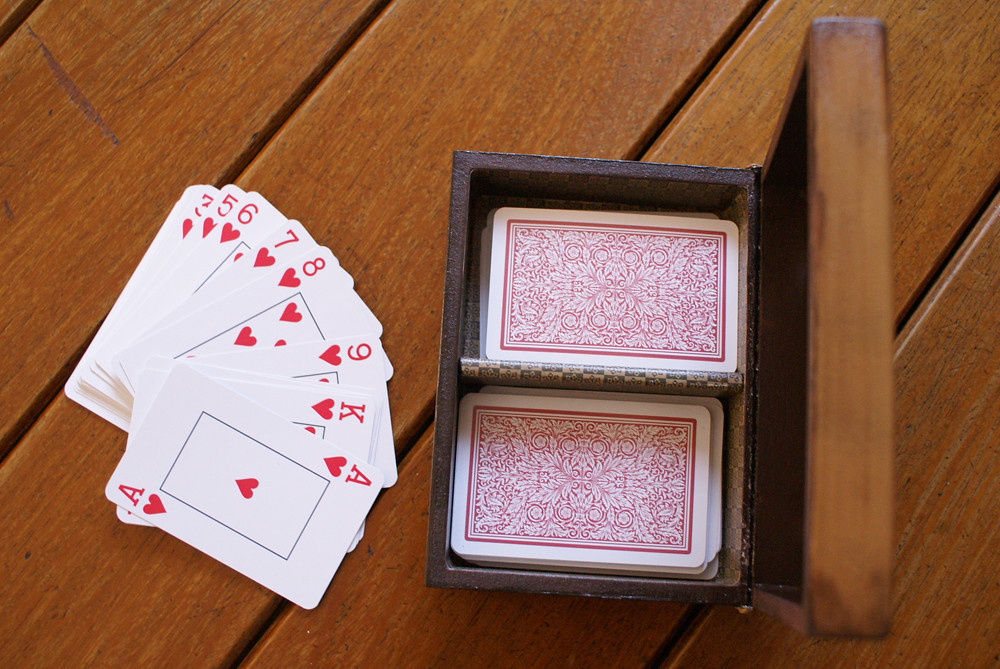The color photograph, taken from a bird's eye view, captures a wooden box designed to store playing cards, resting on a wooden table or decking. The box, crafted from lacquered brown wood with a distinct grain and darkened edges, is open, revealing its two compartments divided by a central partition. Each compartment holds a deck of cards face down, showcasing a red backing with an intricate swirly leaf pattern framed by a white border. 

To the left of the box, several cards from the hearts suit are fanned out face up on the table, displaying the Ace, King, and numbered cards from nine down to six in relative order, though some intervening cards are missing. The faces of these cards are predominantly white, adorned with black-outlined rectangles, red heart symbols in the center, and corresponding ranks in the top left and bottom right corners. The box and cards rest on a surface composed of wooden panels aligned diagonally from the bottom left to the top right, contributing to the rustic aesthetic of the scene.